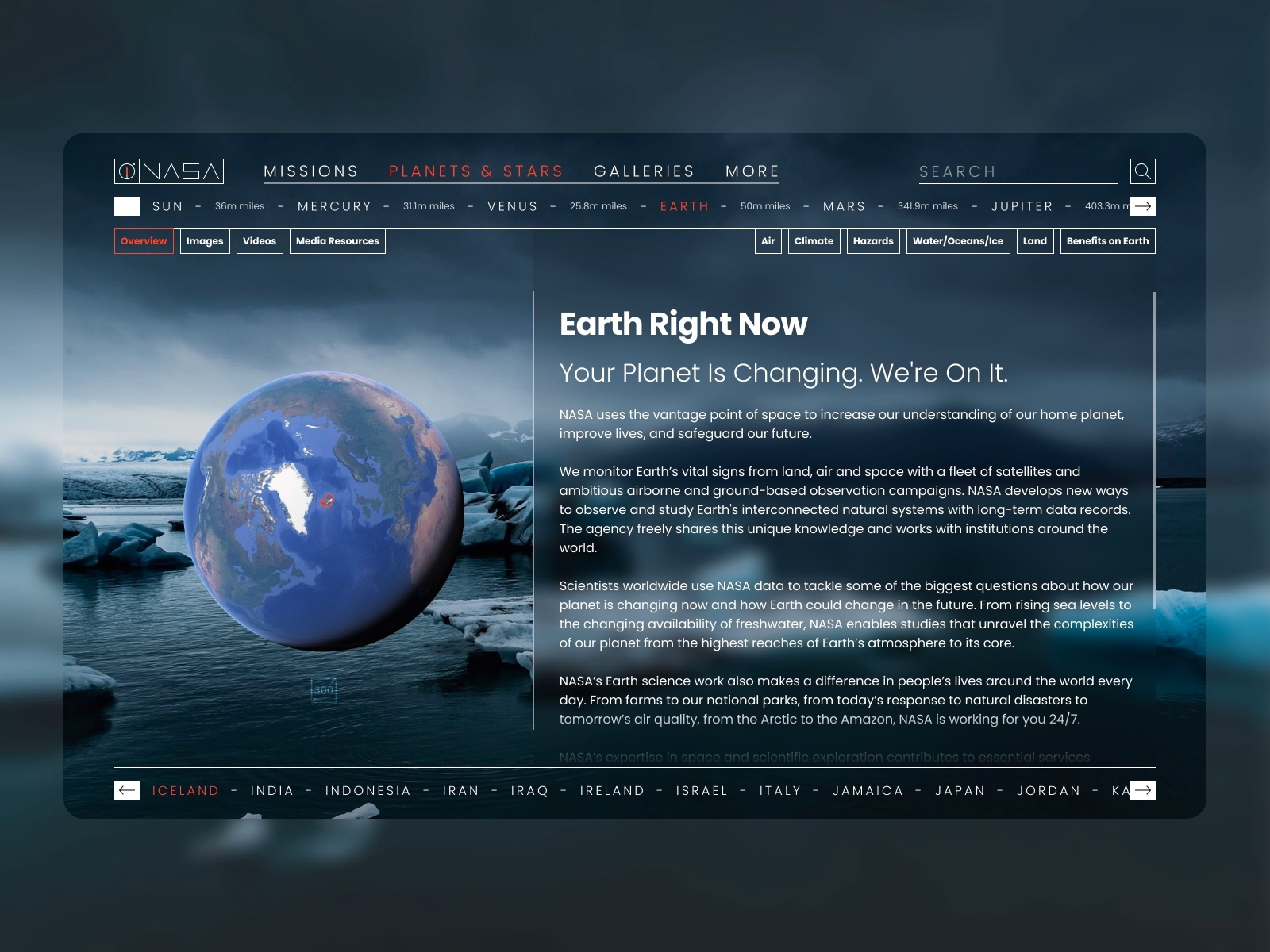The image displays a vibrant NASA-themed interface featuring options such as "Missions," "Planets and Stars," "Galleries," and more. The "Planets and Stars" section is highlighted in orange, indicating it is currently selected. On the right side of the interface, there's a search bar adorned with a magnifying glass icon. Below the search bar, a list of celestial bodies is visible: the Sun, Mercury, and Venus are among them, though the text for some entries is too small to discern. The list includes Earth labeled "50 miles" and Mars labeled "349 miles," suggesting some form of measurement related to distance or data is being displayed. 

The caption beneath reads, "Earth right now, your planet is changing, we're on it." This emphasizes NASA's commitment to using space technology to enhance our understanding of Earth, improve lives, and secure our future. NASA monitors Earth's vital signs via a comprehensive approach involving satellites, airborne missions, and ground-based observation campaigns. Additional information is available, likely providing further details on these initiatives.